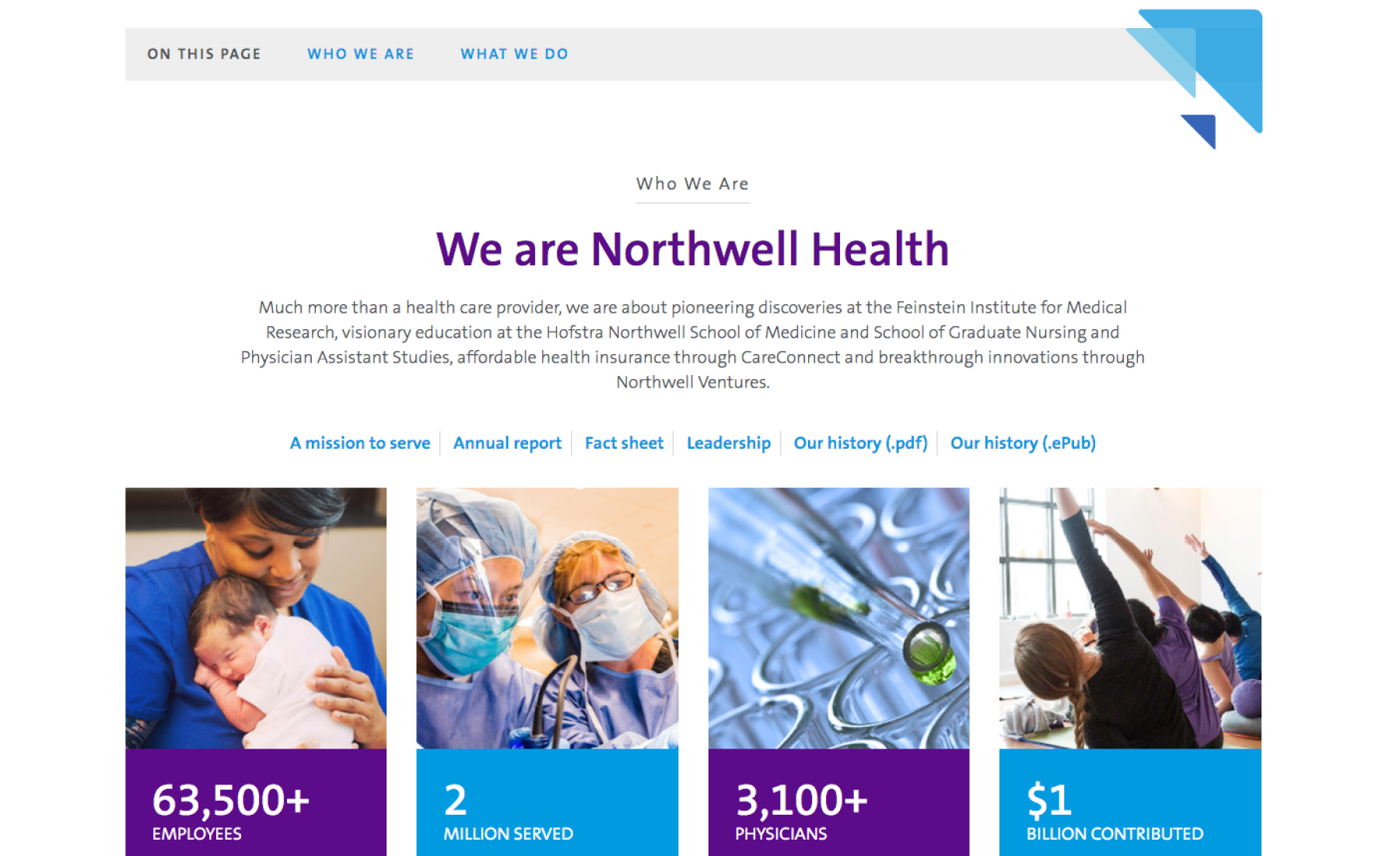At the very top of the web page, a light gray banner features the text "On This Page: Who We Are and What We Do" in gray and blue. Directly beneath this, centered in the main section of the page, bold purple text announces "We Are Northwell Health." Above this headline, smaller text reads "Who We Are," introducing a detailed paragraph below.

This paragraph elaborates that Northwell Health is far more than just a health care provider. It highlights their pioneering discoveries at the Feinstein Institute for Medical Research, visionary education at Hofstra Northwell School of Medicine, Graduate Nursing, and Physician Assistant Studies, affordable health insurance through CareConnect, and breakthrough innovations via Northwell Ventures.

Further down, a series of categories are displayed from left to right in light blue text: "A Mission to Serve," "Annual Report," "Fact Sheet," "Leadership," "Our History in PDF," and "Our History in EPUB."

Under these categories, there are four vertical images arranged side by side. The far-left image shows a woman holding a baby. Next to it, the second image features two women wearing masks. The third image offers a close-up of advanced technology, while the far-right image depicts a yoga class in action.

Below these images, banners in purple and blue present key statistics: "63,500+ Employees," "2 Million Served," "3,100+ Physicians," and "$1 Billion Contributed."